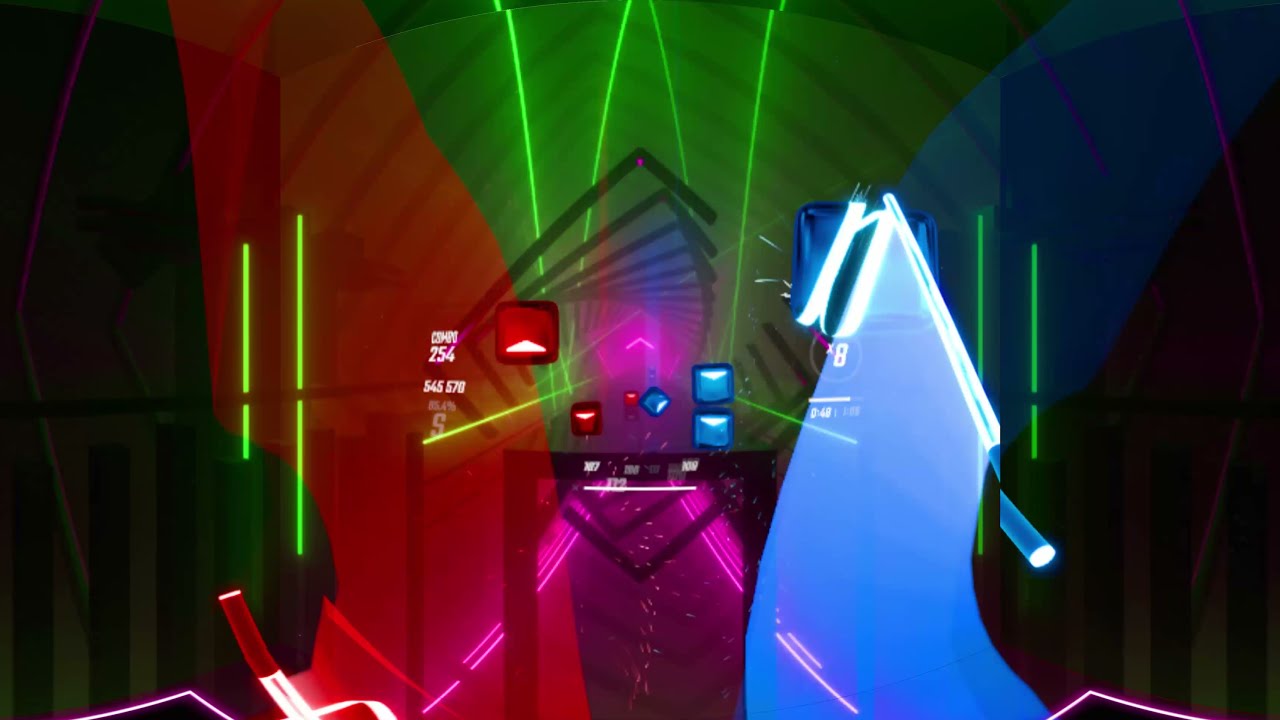This image is a vibrant and detailed in-game screenshot of the VR rhythm game Beat Saber. It showcases a dynamic and colorful scene where the player uses two lightsaber-like wands—a red one in their left hand and a blue one in their right hand—to slice through incoming red and blue cubes that float through space towards them. The left side of the image displays a score of 254 with additional numbers 565 and 570, along with an 'S' denoting a particular ranking or step multiplier. On the right side, it shows a multiplier of 8 and an additional value of 0.4. The background is a dark, futuristic room filled with geometric structures and illuminated by green lasers. The room’s green vertical lights and darker square pillars add to the cyberpunk aesthetic. In the center of the image, there are sparks and motion blurs from the lightsabers, accentuating the action. At the bottom, there’s a pink, road-like path with additional sparks, making the scene vibrant and energetic. The color scheme transitions from dark green on the far left to a swath of red, purple, and green towards the right, culminating in light blue and dark blue before returning to dark green on the far right.